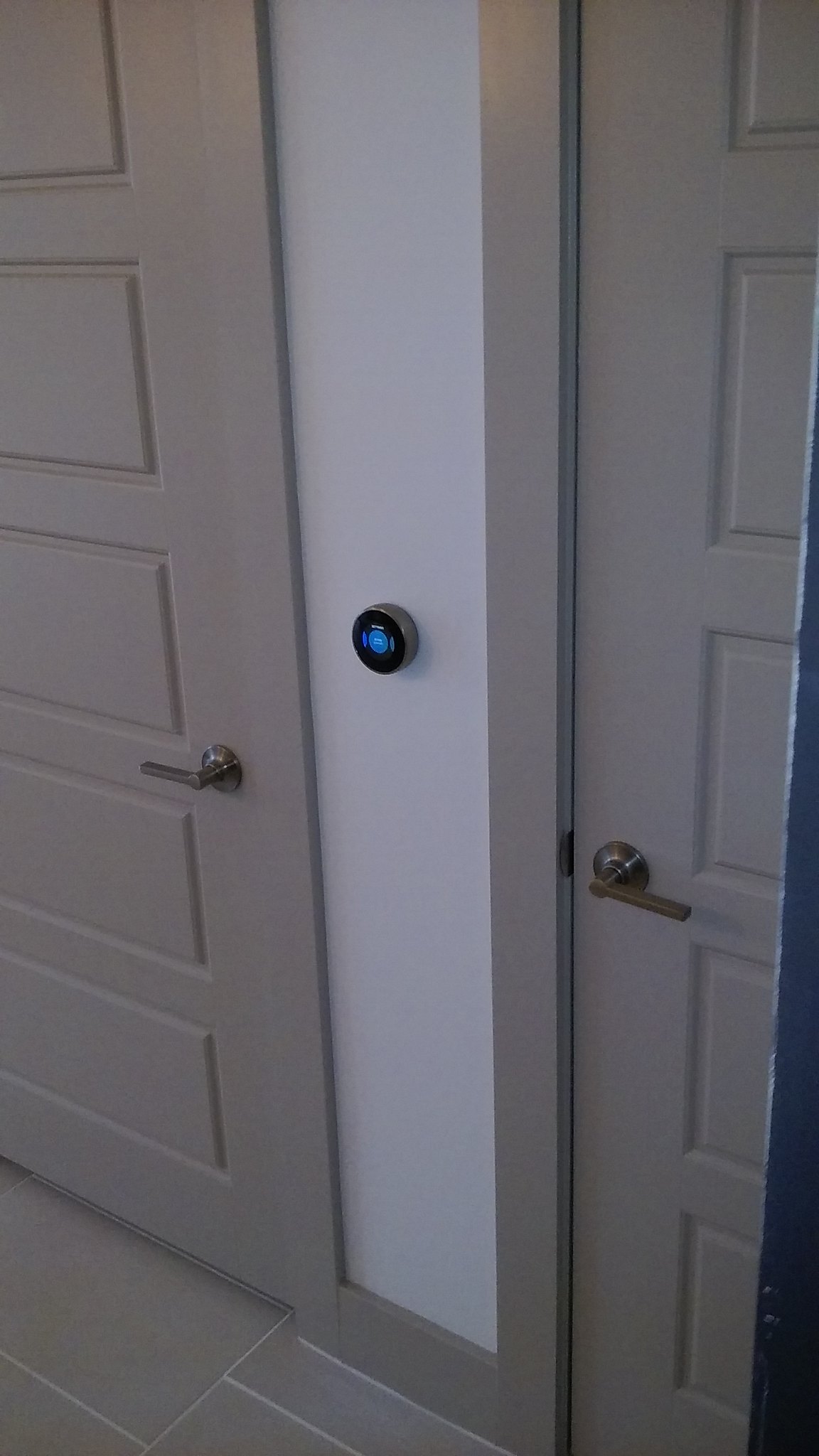This photograph captures a well-composed indoor scene featuring two side-by-side, dove gray doors. Each door is adorned with handles that exhibit a unique blend of bronze and silver hues. Between these doors, there is a slim segment of an off-white wall, which hosts a round digital thermostat with a silver base and a black body displaying a distinctive blue glow at its center. Surrounding the doors is a subtle dove gray trim, harmonizing with the overall color palette.

The floor consists of dove gray tiles accentuated by visible white grout lines, which add a subtle texture to the lower portion of the image. Natural or artificial light reflects softly off the painted surface of the doors, enhancing their sleek appearance. To the far edge of the photograph, a partially visible, dark-colored metal strip catches the eye, hinting at another object just out of the frame. This metal strip shows signs of wear, with some white spots suggesting chipped coating.

The image possesses a slightly grainy texture, yet the details remain clear, contributing to an overall sense of depth and realism.